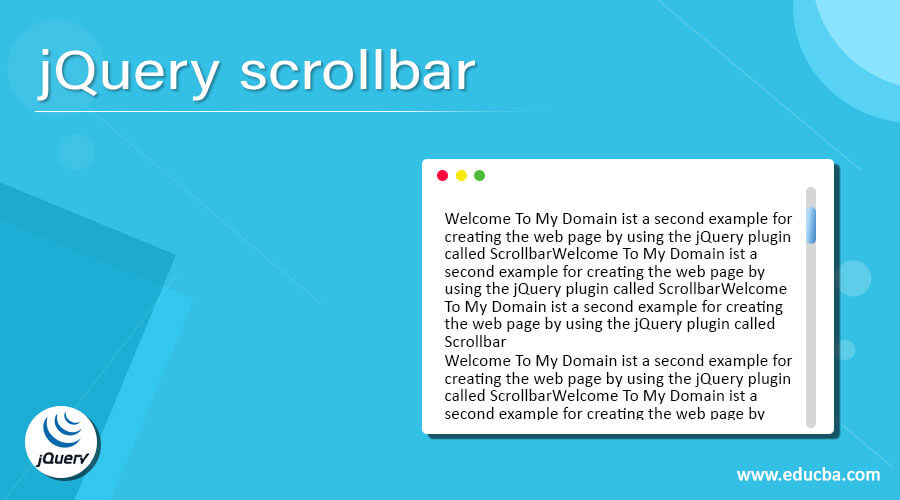A screenshot is displayed with a visually appealing blue background adorned with subtle graphic design elements in the upper right and lower left corners. In the upper left corner of the image, bold white block text reads "JQuery Scroll Bar," accompanied by a faint white underline that adds a clean and modern touch. Dominating the lower right corner is a prominent white text box containing a repetitive, placeholder message: "Welcome to my domain. A second example for creating the webpage by using the JQuery plugin called scrollbar. Welcome to my domain. First, a second example for creating the webpage by using the JQuery plugin called scrollbar. Welcome to my domain." The text is clearly intended to demonstrate examples of the JQuery scrollbar plugin in action. To the right side of the text box, there is a vertical scroll bar colored gray, with a distinctive blue pull-down button, indicating the ability to scroll through the extensive text. The overall design effectively showcases the usage of JQuery plugins to enhance web content.